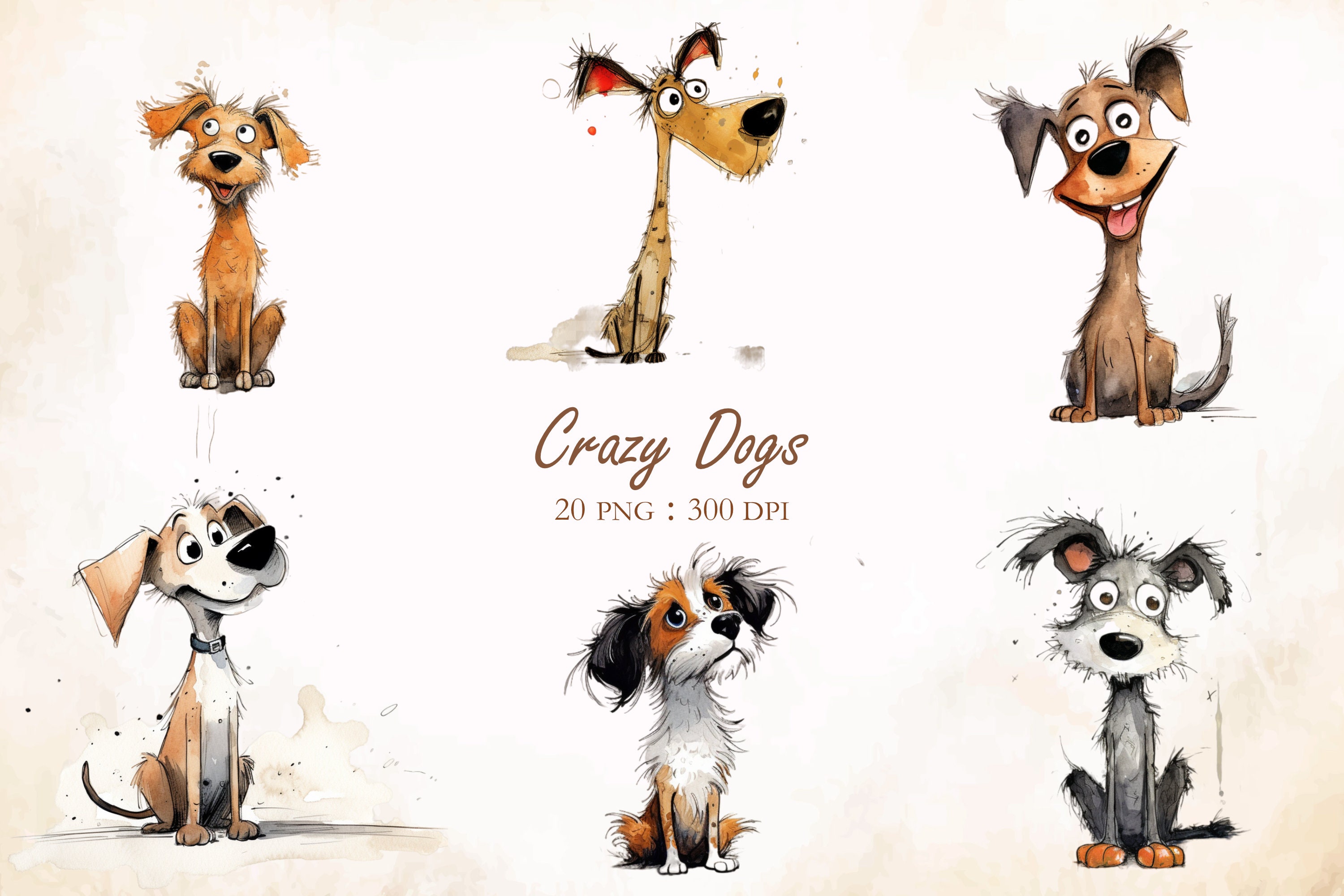In this beautifully illustrated watercolor-style image, set against a white background with light brown, scroll-like watermark accents along the edges, six distinct dogs are depicted sitting on their hindquarters, each showing different expressions and facing various directions. At the center of the image, in elegant script, it reads "Crazy Dogs," followed by "20 PNG, 300 DPI" in standard print beneath it. On the top row, starting from the left, a light brown dog with floppy ears sits happily looking up to his right. Next to him, a skinnier yellow dog with black, perky ears gazes off to his left with a disheveled, neutral expression. The third dog on the top is a fluffy brown dog with perky ears, joyfully looking straight ahead with his tongue out, seemingly wagging his tail. On the bottom row, from left to right, a brown dog with white markings on his face and belly, wearing a blue collar, smiles up to his left. In the middle, a dog with a white face, brown markings around his eyes and legs, and black floppy ears appears slightly sad, gazing up to his left. The last dog on the right, distinct with his gray and white fur, looks slightly off-center to the left with a neutral expression. This charming collection of sitting dogs captures a range of emotions and adds a lively, whimsical touch.